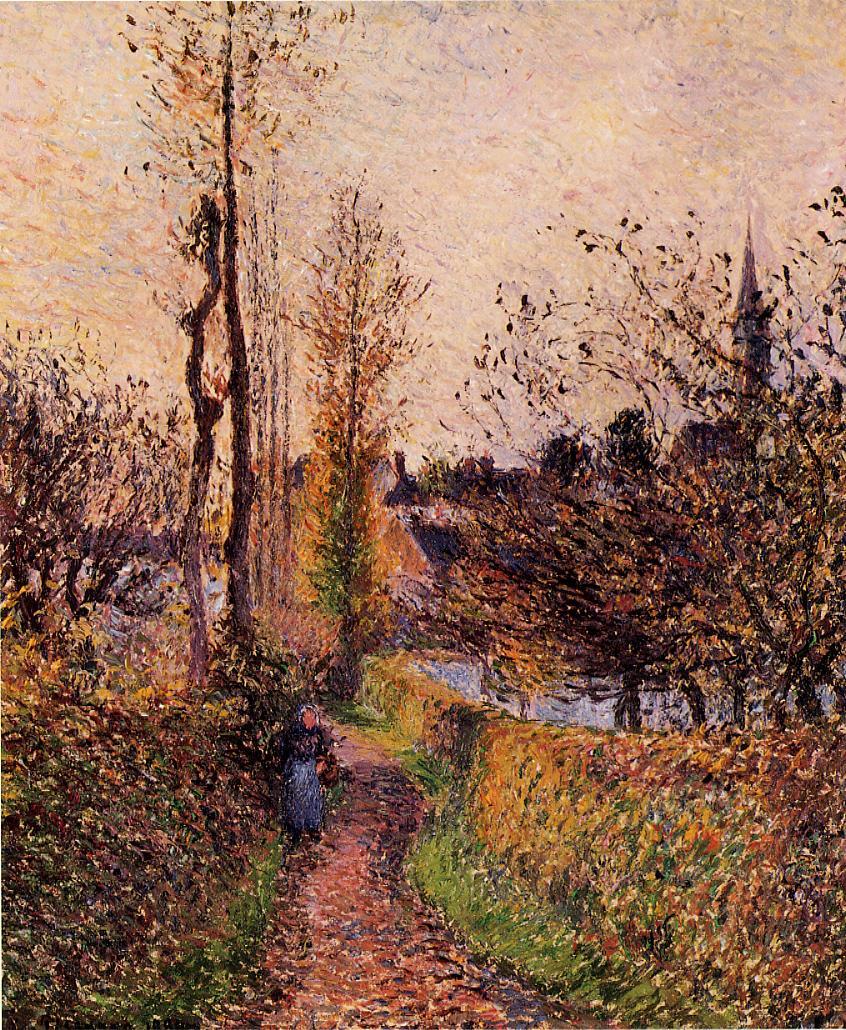This painting, rendered in an impressionistic style with small to medium brushstrokes, captures a scenic autumn landscape. A woman, discernible by her black top and blue dress, walks towards the viewer along a winding, reddish-brown dirt path strewn with leaves. This path cuts through a lush setting with well-trimmed green and yellow bushes on either side. To her right, a riverbank hints at the meandering presence of a stream or lake. Flanking the trail are barren tree trunks and a mosaic of trees with sparse orange foliage, emphasizing the fall season. The background reveals a quaint village with a prominent church steeple rising against an evocative sunset or sunrise sky. The painting's rough, muted tones and lack of fine detail create a beautifully immersive scene that becomes clearer from a distance, drawing the viewer into its rustic tranquility.